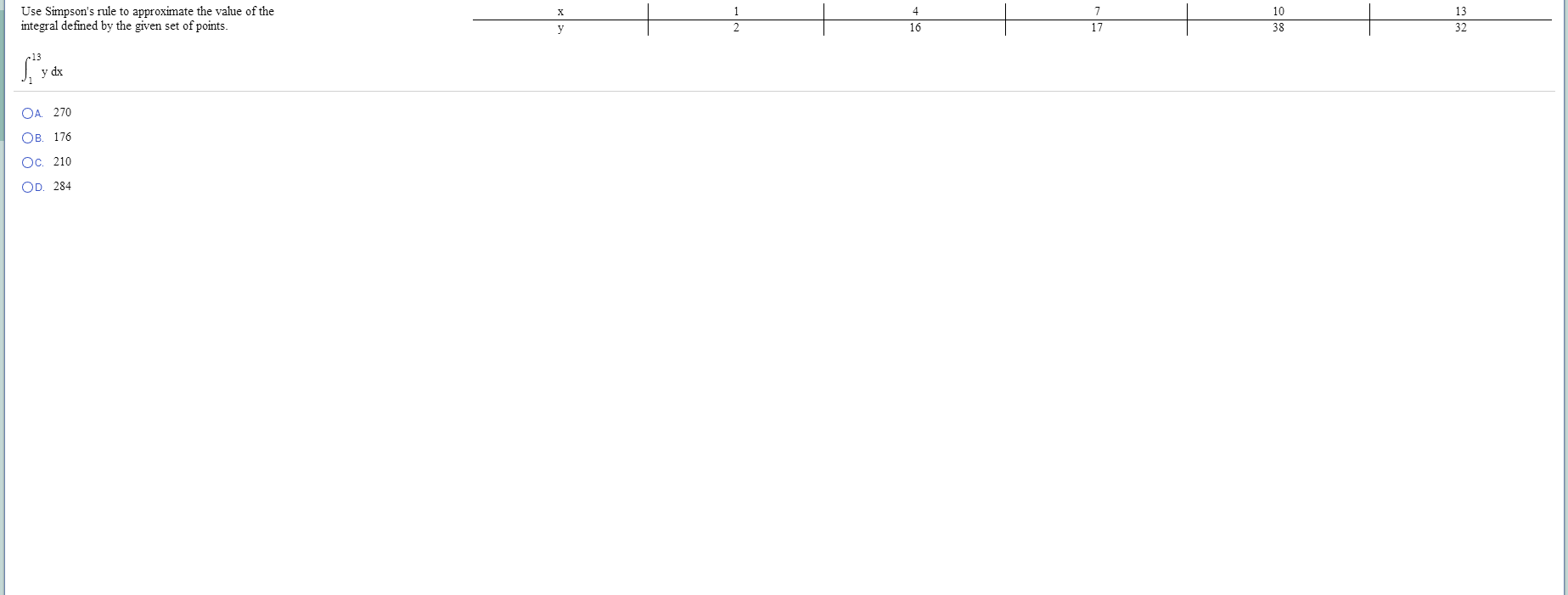In the top left corner of the image, there is a mathematical problem involving Simpson's Rule for numerical integration, labeled "Simpson's Rule 2." The integral to be solved is expressed as ∫ from 1 to 13 of y dx. To solve this integral, specific points are provided on the x-axis (1, 4, 7, 10, 13) and corresponding values on the y-axis (2, 16, 17, 38, 32). The problem offers four multiple-choice options for the integral's value: 

- a) 270 
- b) 176 
- c) 210 
- d) 284

The x-axis is segmented and labeled at intervals of 1, 4, 7, 10, and 13. These segments are visually represented as hollowed-out sections aligning with their corresponding y-values. Simpson's Rule, requiring these specific points, suggests the area under the curve is divided for calculation.

On the far left, there is a solid gray vertical divider that acts as a boundary for the problem's layout. The clarity of sections and proper labeling are essential to solving the equation using Simpson's Rule, by methodically summing areas under each segment of the curve.